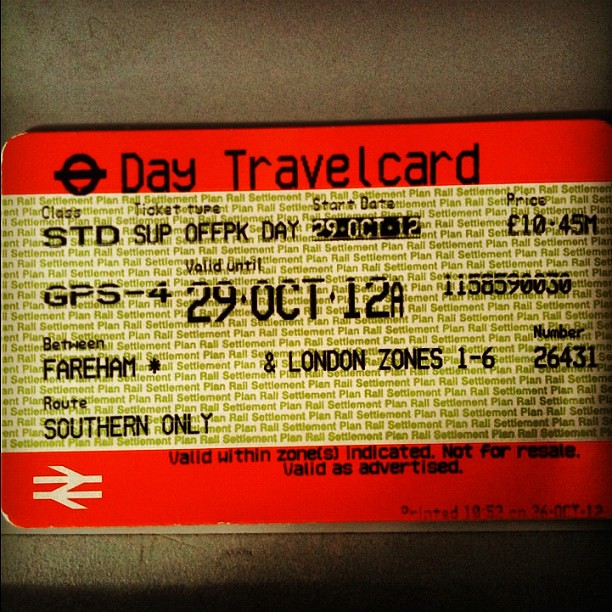The image depicts a rectangular ticket with rounded edges, set against a brown background. The ticket features prominent red bars at both the top and bottom. The top red bar displays a black icon of a circle with a line through it accompanied by the text "Day Travel Card." The bottom red bar also includes a logo consisting of white crisscrossing arrows to the left, followed by the text "Valid within zones indicated. Not for resale. Valid as advertised."

The central section of the ticket is white with green watermark text, possibly displaying the "Settlement Plan Rail" repeatedly to prevent forgery. The primary details are printed in black font in the middle. Key information includes the class "Standard," ticket type "SUP" and "OFFPK Day," and the date range "Start Date: 29 Oct 12" with validation until "29 Oct 12A." Additionally, it lists a price, a unique GPS identifier, the validity zone "Fairham Star to London Zones 1-6," and a route specified as "Southern only."